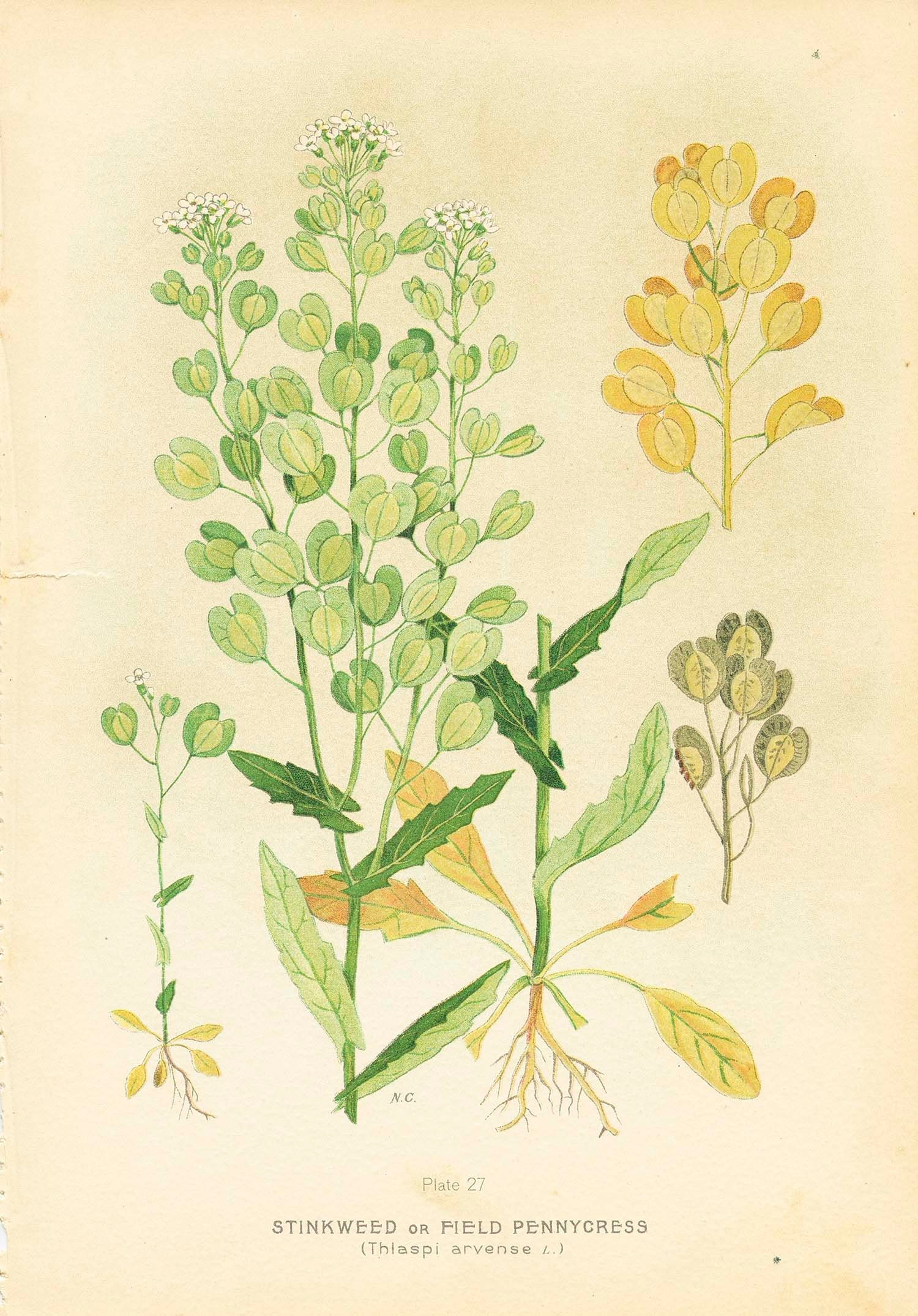The image depicts a detailed botanical illustration scanned from an old, yellowed piece of paper that shows various specimens of a plant known as Stinkweed or Field Pennycress, with its scientific name, Thlaspi arvense, annotated at the bottom as "plate 27 NC." The paper appears aged, with a small rip on the left side and a black dot at the bottom right. The artwork showcases different stages and parts of the plant, including a central large branch that is light green with many elongated leaves and white flowers at the top. The top right corner of the image highlights a version of the plant with yellow flowers and stems, while another part shows the plant's leaves in black and orange. The detailed illustration makes it clear that the same plant is represented in different conditions and growth stages.